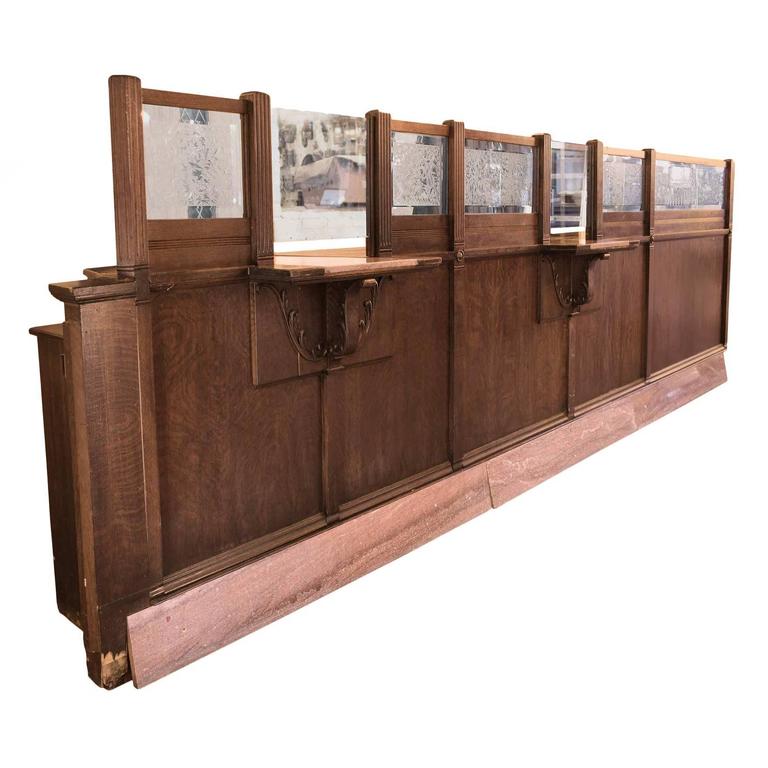The image depicts a vintage bank teller window, an antique wooden counter stand likely pulled directly from an old bank. The structure is fixed to the ground, showcasing a long countertop made of mahogany wood. It features seven glass panes bordered by wood for stability; the top half of the image prominently displays these panes, which have some design allowing one to see through them. In this setup, there are two primary teller windows, the second and fourth panes, equipped with protruding wooden trays or writing lips where people could place items or write checks. These two windows don't have a wooden top border, making them unique compared to the other panes. The background is white, giving an indoor feel to the scene, emphasizing the potential auction or display context of this antique piece. Overall, this piece recalls an old-time bank or casino counter, complete with the traditional elements one would expect from such vintage furniture.